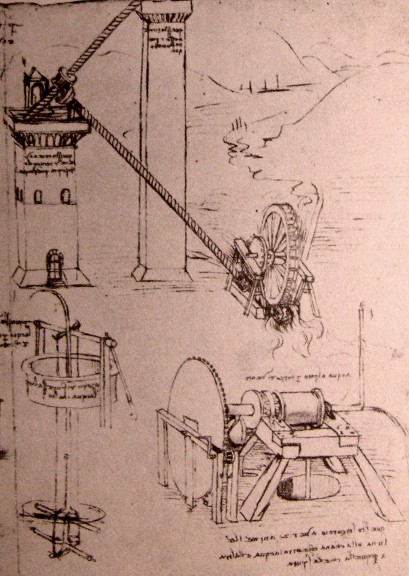The image appears to be an intricate, historical blueprint reminiscent of Leonardo da Vinci's work, depicting a complex machinery system. The sketch, likely created with pencil or ink, is detailed in black on a brownish-orangish paper, exuding a distinctly aged feel. The drawing features multiple interconnected mechanical elements, including wheels, gears, and perhaps a saw. A river flows through the scene, possibly powering the machinery, which includes devices resembling water wheels, pumps, or motors. In the background, faintly sketched mountains and hills provide a subtle landscape context. Two towers, connected by ropes and linked to a mill, dominate the upper portion of the image. Additionally, the sketch is accompanied by illegible writing in a foreign script, further enhancing its antiquated and enigmatic nature.